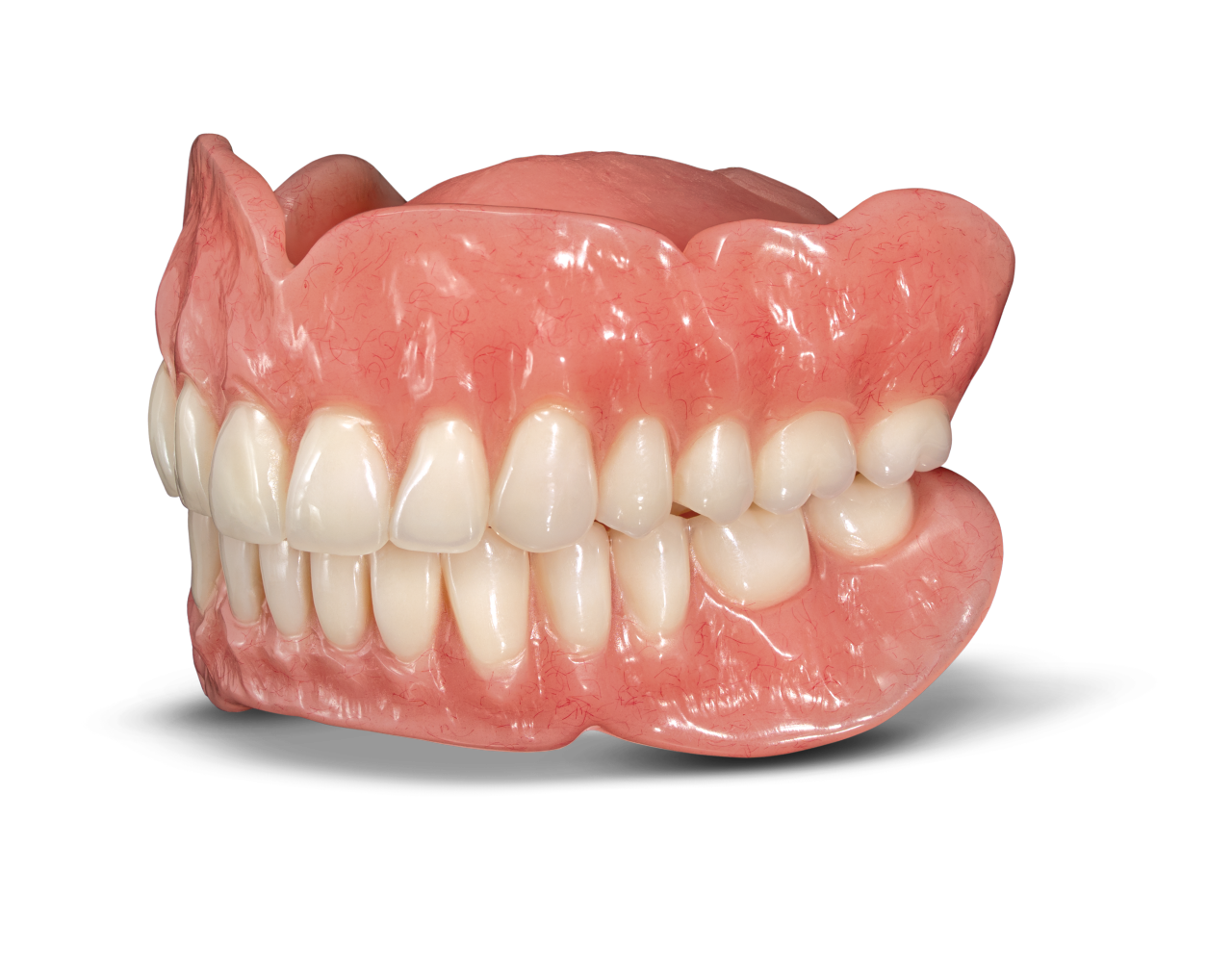The image features a detailed and realistic pair of dentures with complete upper and lower sets of teeth and gums. The teeth are remarkably straight, white, and well-aligned, suggesting they are in pristine condition. The gums are a vivid pink, uneven in contour with small cliffs and dips, enhancing the lifelike appearance. The gums also appear to be reflective, which, along with the glossy texture of the teeth, implies that the dentures are likely made of hard plastic or a similar material. The dentures are positioned such that the two front teeth are tilted towards the bottom left of the scene. The background of the image is entirely white and featureless, giving it a clean, clinical aesthetic, with a noticeable shadow underneath the dentures, emphasizing their three-dimensional form.